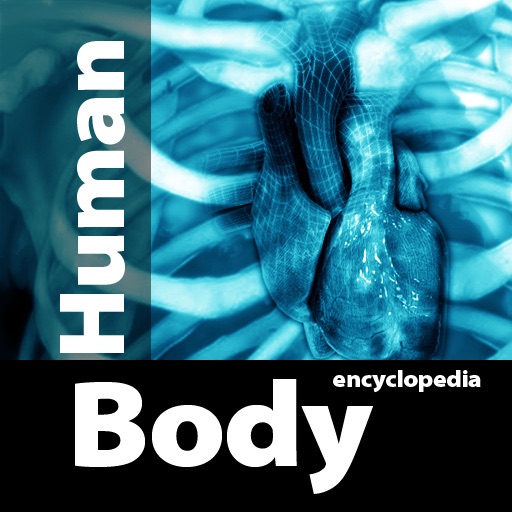The image appears designed as a magazine cover, likely health-related, featuring a computer-generated, x-ray-like rendering in shades of blue. The primary visual content displays a human ribcage encasing a glossy, wet-looking heart, with arteries visible, set against a deep blue backdrop. Overlaying the image, the words "human body encyclopedia" are arranged vertically on the left and horizontally at the bottom. The text "human" is presented sideways in white within a translucent black-grey box, while "body encyclopedia" is written in blocky, white 90s-style fonts on a solid black bar at the bottom, with "body" being the most prominent word. The overall composition is placed within a square frame, and the interplay of black, white, and blue hues dominates the visual experience, evoking the look of an x-ray film.